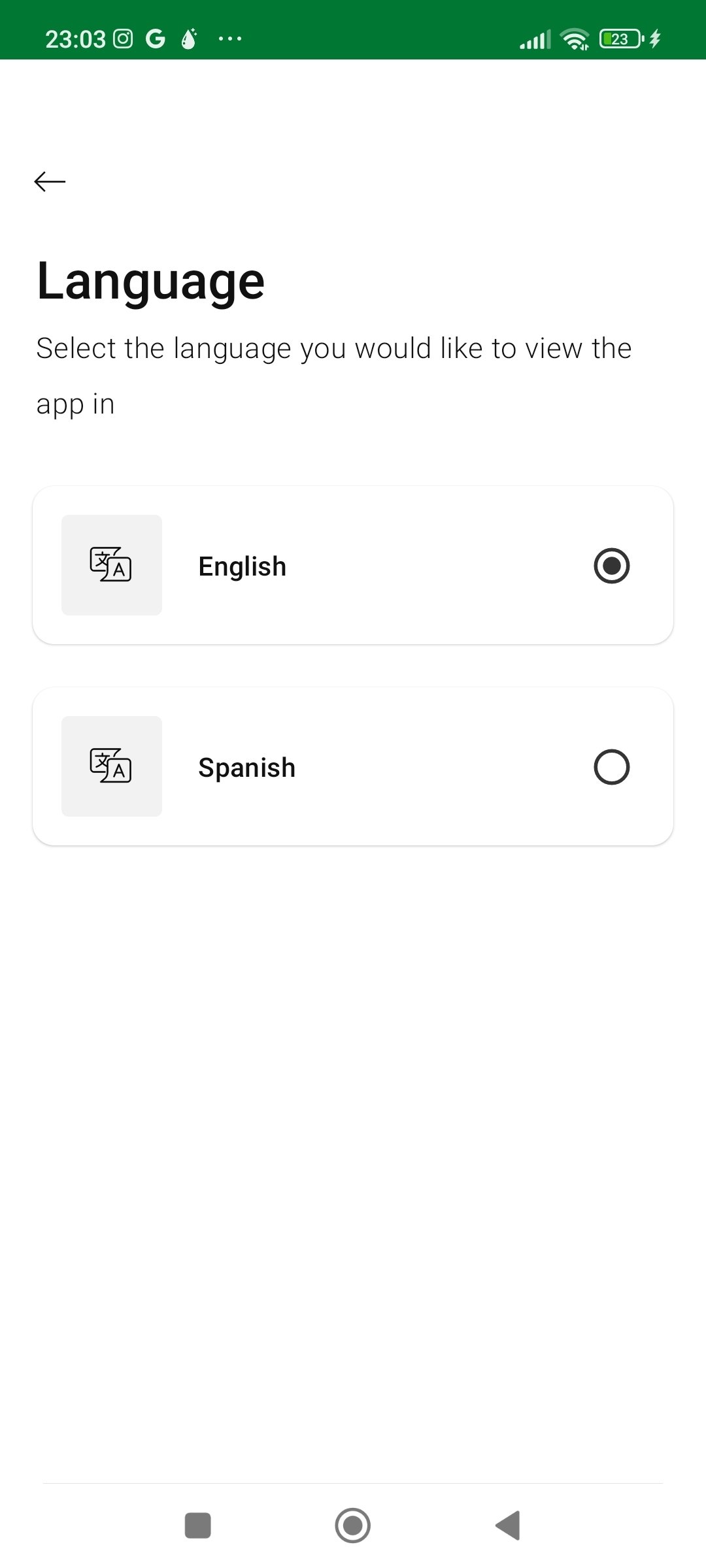The screenshot captures a language selection screen within a mobile application, presented with a clean and straightforward interface. The top section of the screen features a green status bar displaying the current time as 23:03, along with standard icons for signal strength, Wi-Fi connectivity, and battery life at 23%, including a charging indicator.

Below the status bar, the title "Language" is prominently displayed, accompanied by a subtitle that prompts users to "Select the language you would like to view in the app." Two language options are presented: "English" and "Spanish."

The "English" option is marked with a check mark, indicating it is the currently selected language. Both language options feature a small speech bubble icon containing the letter "A" and a star, likely symbolizing the language settings.

At the bottom of the screen, the familiar Android navigation icons—a square, circle, and triangle—are visible, ensuring easy navigation. The overall layout is minimalist, emphasizing user-friendly navigation and a clear choice between the two available language options.